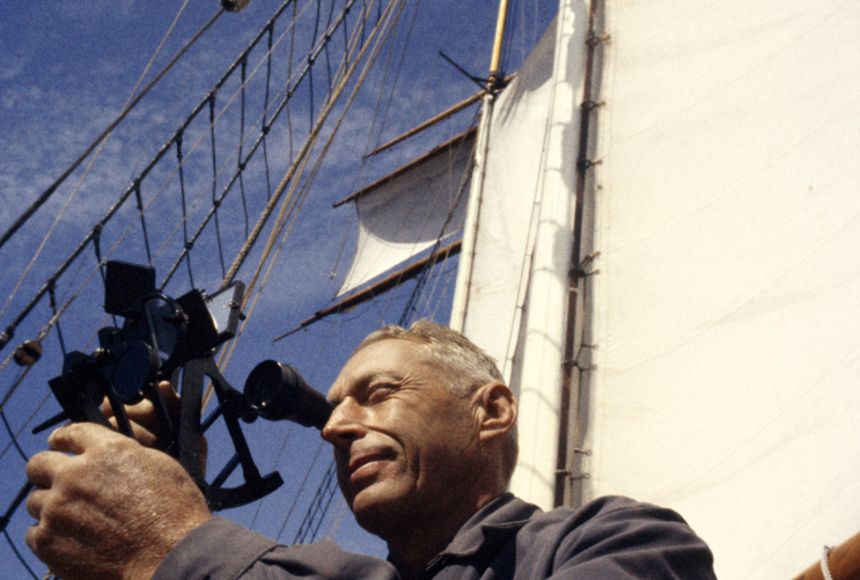The image appears to be a colorized, vintage photograph of an older man with thinning, gray hair, standing on an antique, multi-sailed ship. He is dressed in a dark gray button-down, long-sleeved collared shirt or jacket. The man is facing the left side of the image, holding a black nautical telescope up to his right eye. This telescope features a distinctive square mirror on top, suggesting it is a specialized navigating tool. The scene captures the man’s hands as they hold the device, indicating he may be demonstrating its use. The background reveals the ship's rigging and a large white mast with numerous ropes and at least one rope ladder extending upward. The sky is blue with thin, white clouds. This looks like a professional photograph, possibly of a famous individual or for a magazine article, emphasizing the expertise and vintage ambiance of the setting.